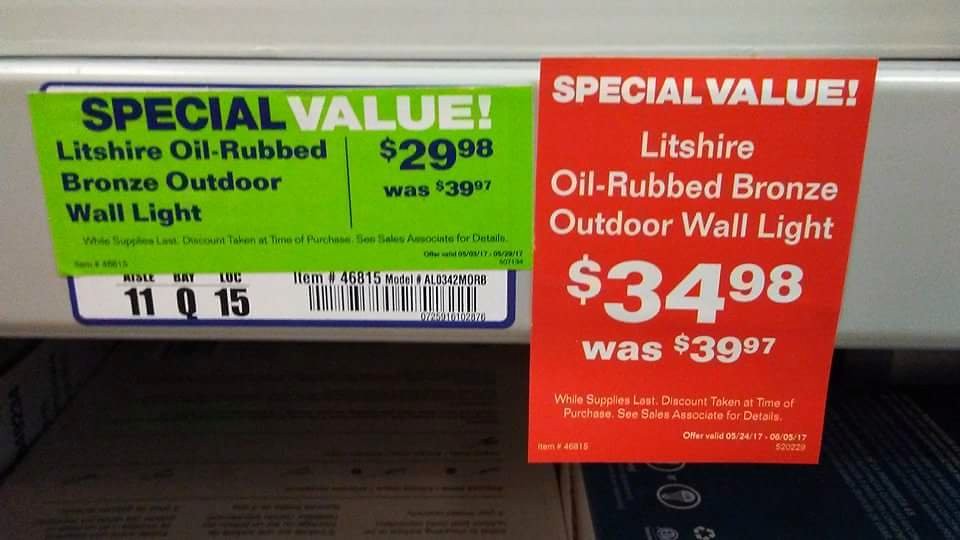This photograph captures a close-up of the price tag attached to the bottom of a light gray metal shelf in a store. Just below this shelf, another shelf with some boxes is partially visible. The primary price tag in view is a sticker affixed directly onto the metal shelf, featuring a light blue outline and a white background, partially obscured by a barcode. On top of this tag, there's an additional lime green sticker with blue and white text, advertising a special value offer: "Light Shire Oil Rubbed Bronze Outdoor Wall Light $29.98 was $39.97." To the right of this sticker, another price tag in red with white font echoes the same information as the lime green sticker.